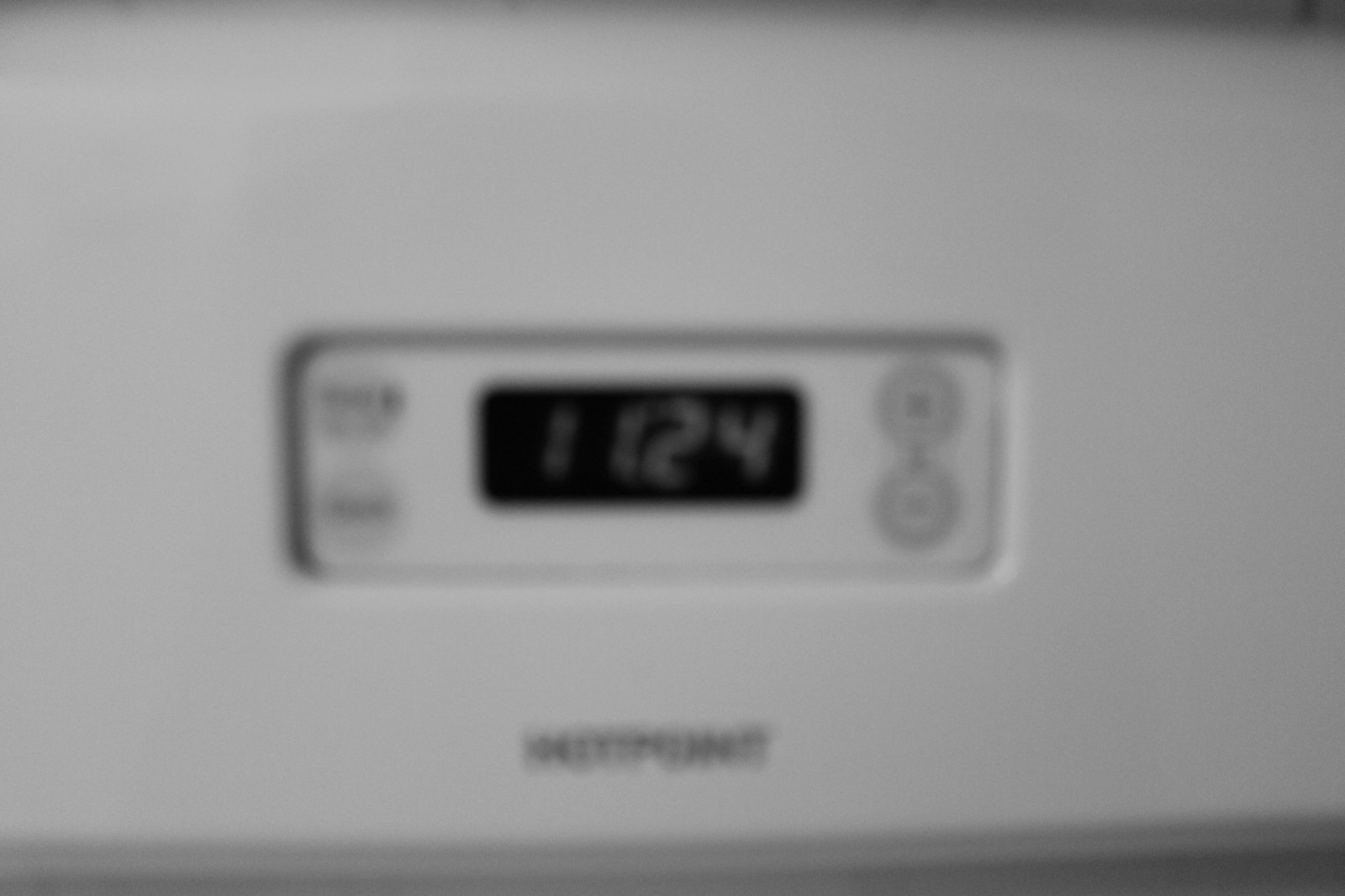This image depicts a close-up view of the top section of a white, enamel metal oven. Though the photo is blurry and slightly out of focus, it reveals a recessed black triangular area in the center of the oven's interface. At the heart of this triangle, an LCD screen displays the current time, which reads 11:24. The ambiguity of the time—whether it is morning or evening—adds a layer of curiosity. Flanking the LCD screen on either side are two touch screen buttons, which, though illegible due to the blurriness, suggest interactive controls. Below the recessed area, the brand name of the oven is printed in black font, but it too remains unreadable in the photograph.